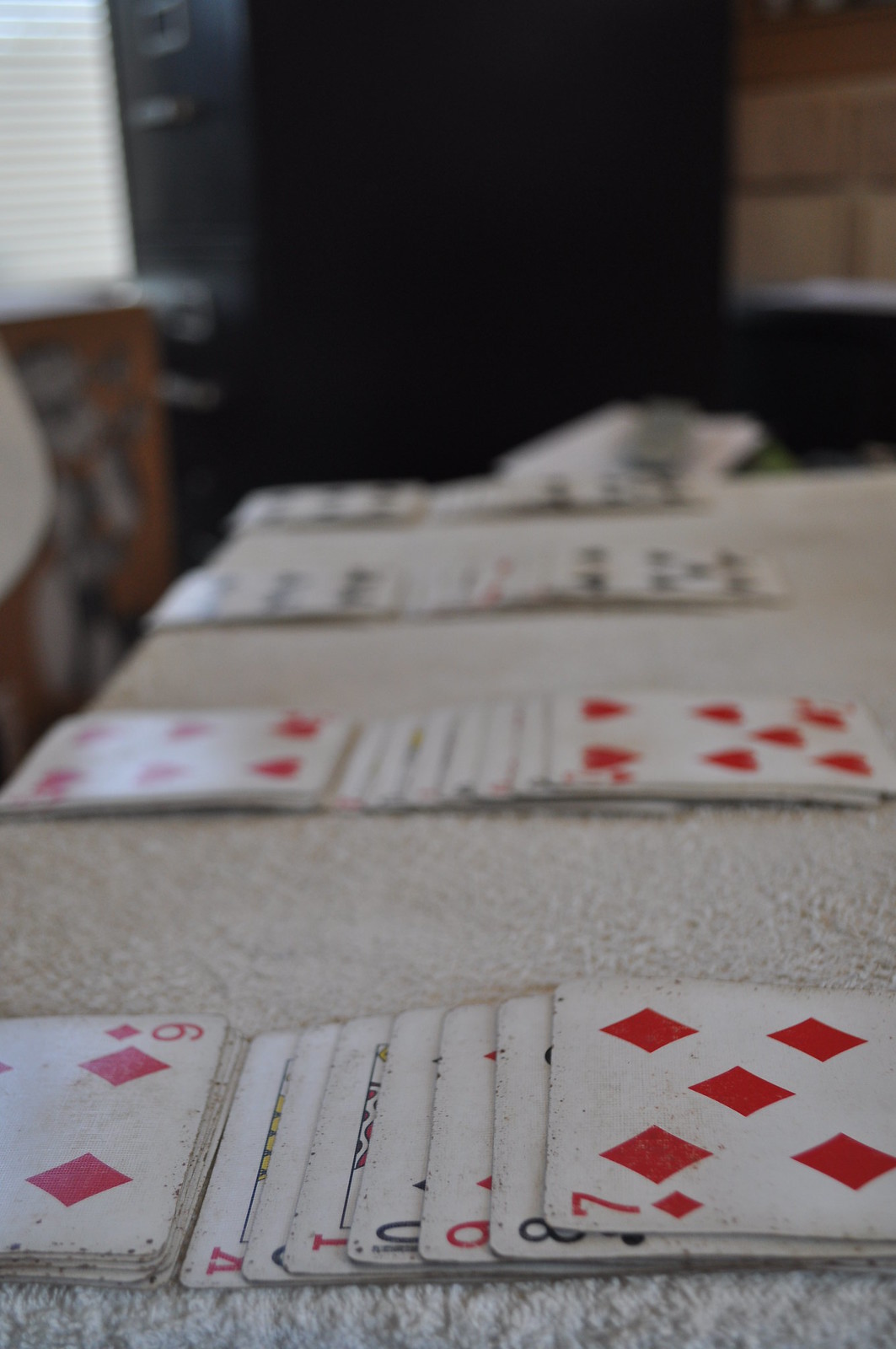In this color photograph, some areas are slightly blurry and out of focus. However, the foreground features a prominently sharp image of a table adorned with a beautiful white lacy tablecloth. At the bottom of the photograph, a spread of playing cards is visible, including the six of diamonds, seven of diamonds, and partially obscured cards such as the king, ten, queen, and jack.

Towards the middle of the image, another stack of cards is similarly laid out but remains unreadable due to the blur, with visible red cards that appear to be hearts and diamonds. Further back, more cards are scattered, these ones being black cards, though their details are also too blurry to discern. 

In the far background, a large, dark-colored bookshelf is partially visible, adding depth to the scene. On the left side of the image, there is a window with Venetian blinds partially covering it, allowing a glimpse of light into the room.